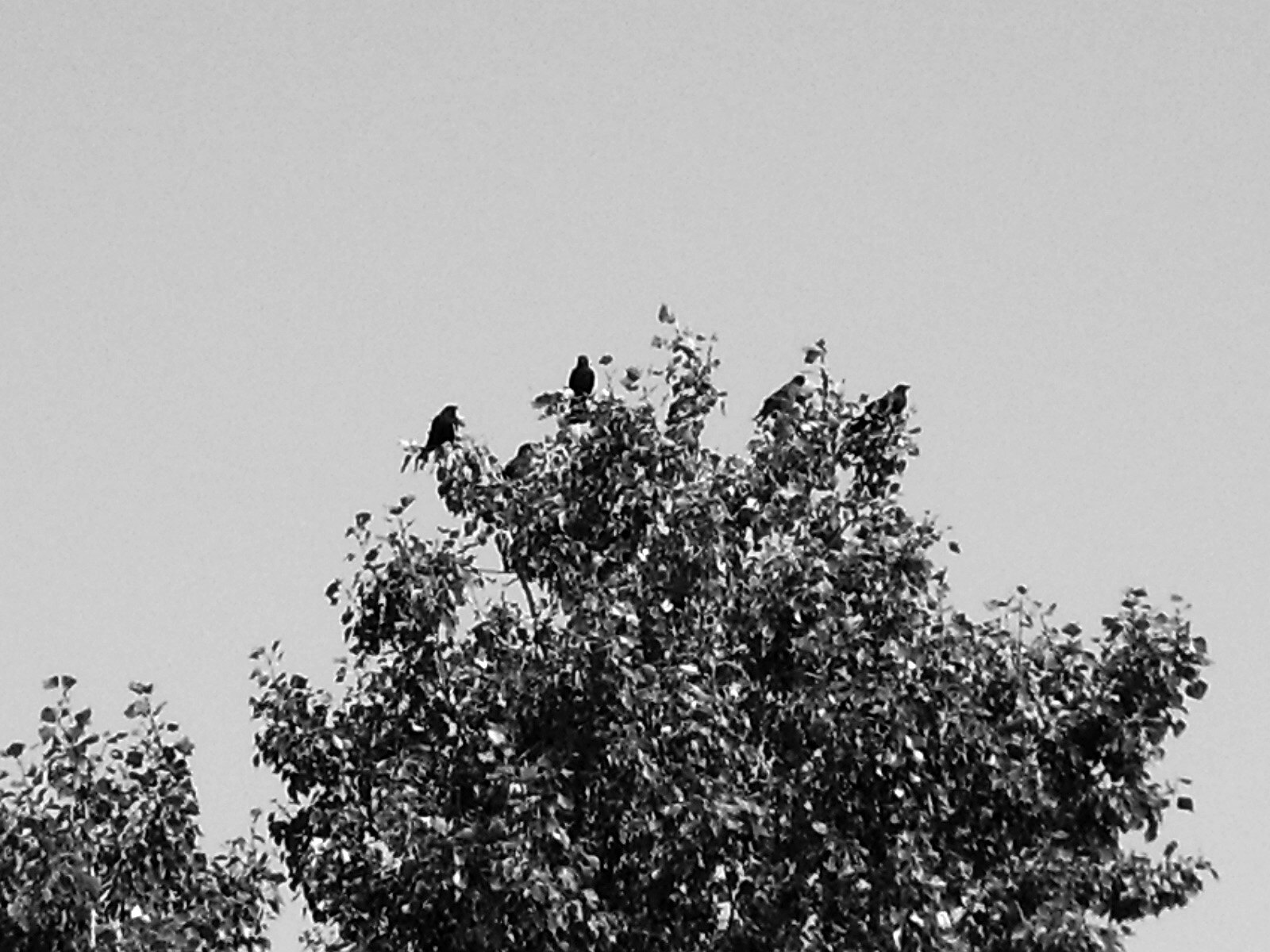In this black and white photograph, the top fourth of a tall, leafy tree dominates the scene, with a smaller tree appearing in the left-hand corner. The dense foliage obscures the trunks of both trees. At the highest point of the main tree, four large birds perch prominently, their dark, unmarked shapes stark against the gray sky, which results from the monochromatic setting. The leaves, large and full-shaped, suggest the tree might be a maple. The angle of the shot implies the photographer stood 10 to 15 feet away, aiming the camera upward to capture this serene, elevated view of nature.